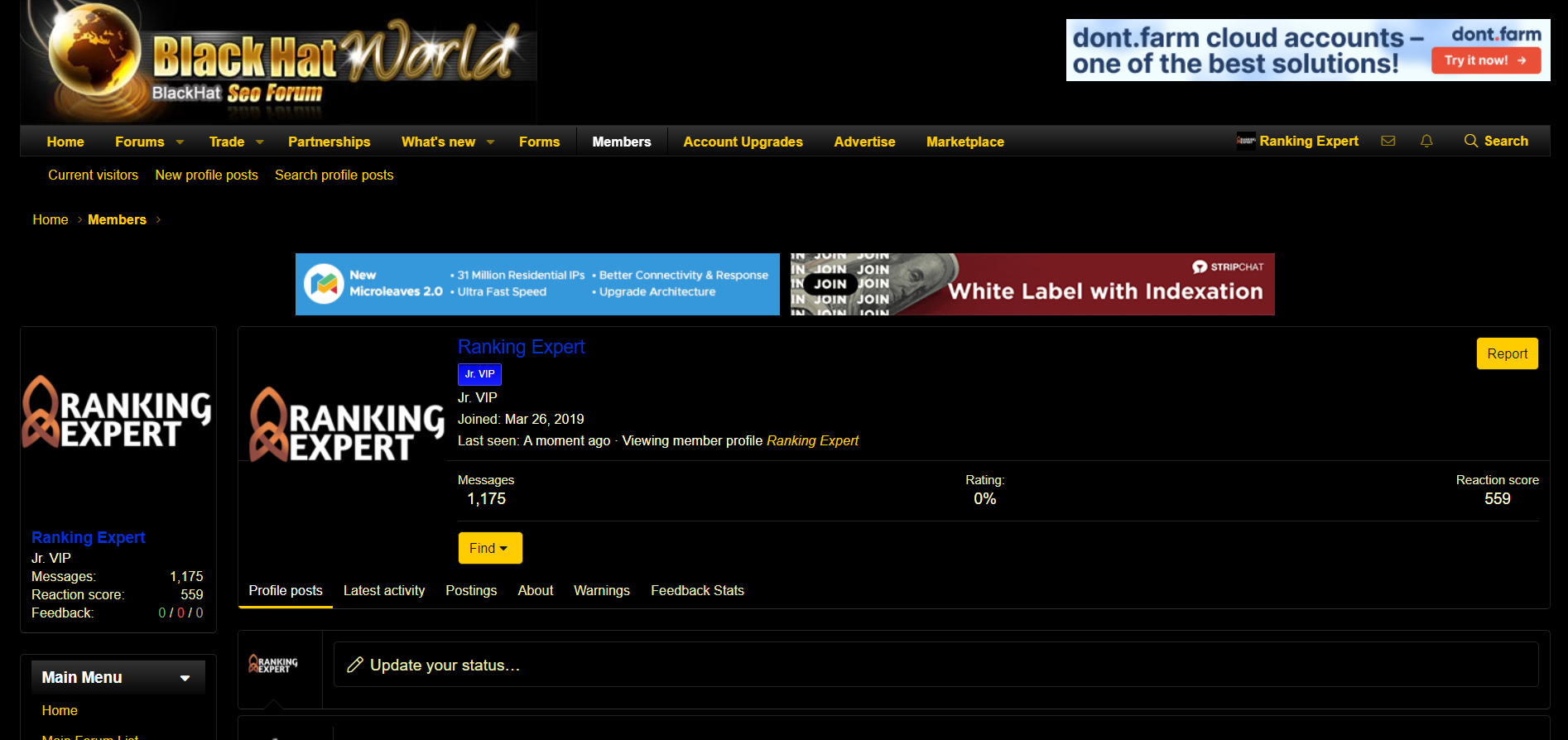The image features a black background. At the top center, there is a golden, illuminated globe displaying the continents, giving off a subtle glow. To the side of the globe, elegant gold text reads "Black Hat." Below it, in a larger, more ornate font, the word "World" is prominently displayed, with sparkling light effects surrounding it. Underneath, the caption "Black Hat SEO Forum" is clearly visible.

On the top right corner of the image, there is a banner with a bright red background and white text. The banner reads: "NC Cloud Background - don't.farm, cloud accounts, one of the best solutions, don't.farm, try it now."

Below this section, the navigation menu is listed in gold text with the following options: Home, Forums, Trade, Partnerships, What's New, and Forums again. The word "Members" is in white text, followed by other options in gold: Account Upgrades, Advertise, Marketplace.

To the right of these options, the text "Ranking Expert" is present. There are also icons representing an email envelope, a notification bell, and a magnifying glass for search functionality.

Further down the image, there are two banners - one blue and one red. Below these banners, the text "Banking Expert" appears twice. Additionally, there is a numeric message displayed as "$1,125" accompanied by a gold square with the text "Find" inside it.